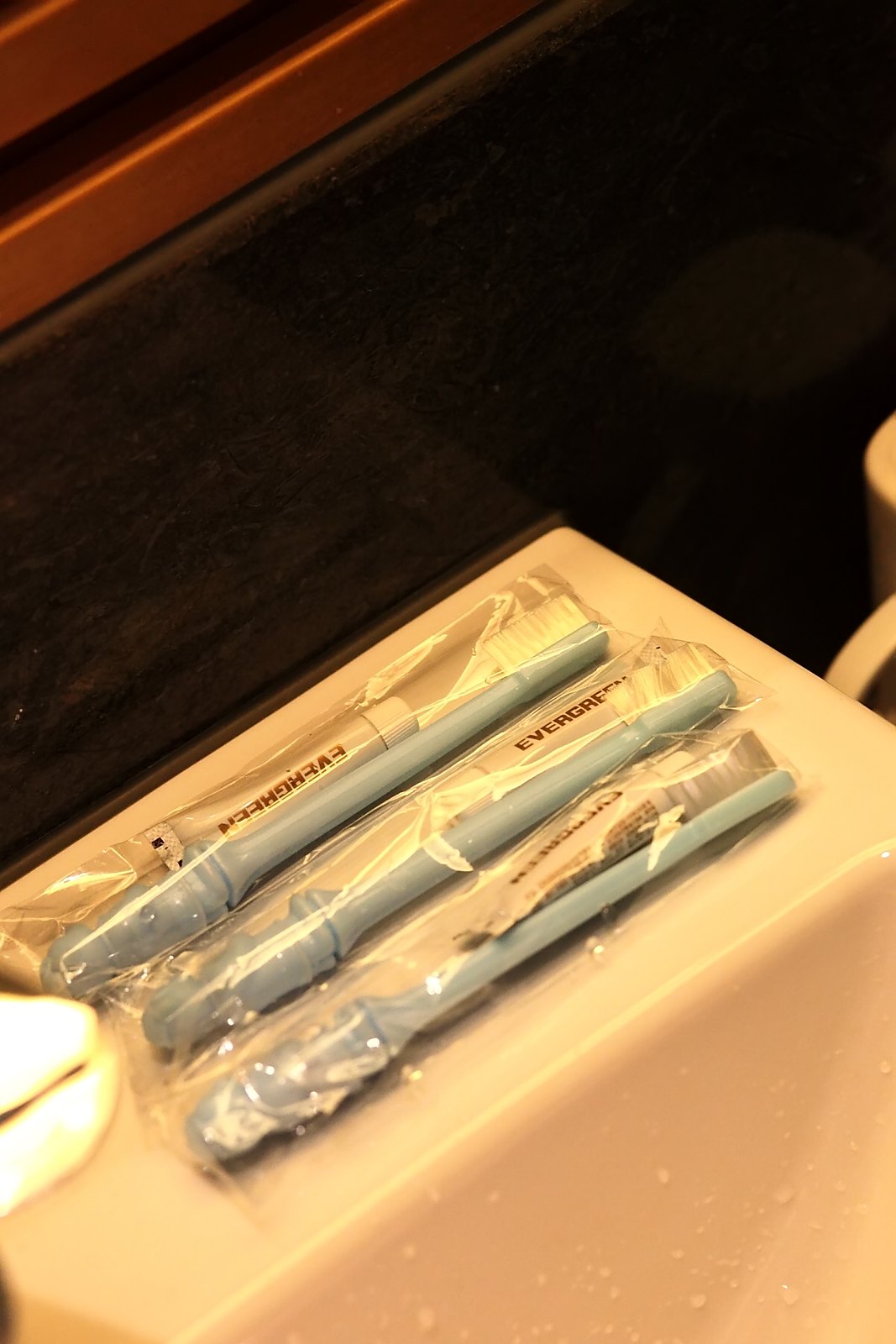The photograph depicts three travel packages of toothbrushes, each containing a sky blue or mint green handled toothbrush with soft bristles on one end and a protective cap on the other. Both the toothbrush and a white tube labeled "evergreen," presumably toothpaste, are sealed inside clear plastic packaging. These packages are positioned on the edge of a white porcelain sink, which has visible water droplets. The surrounding surfaces include a black tile area and hints of red and yellow elements in the background.